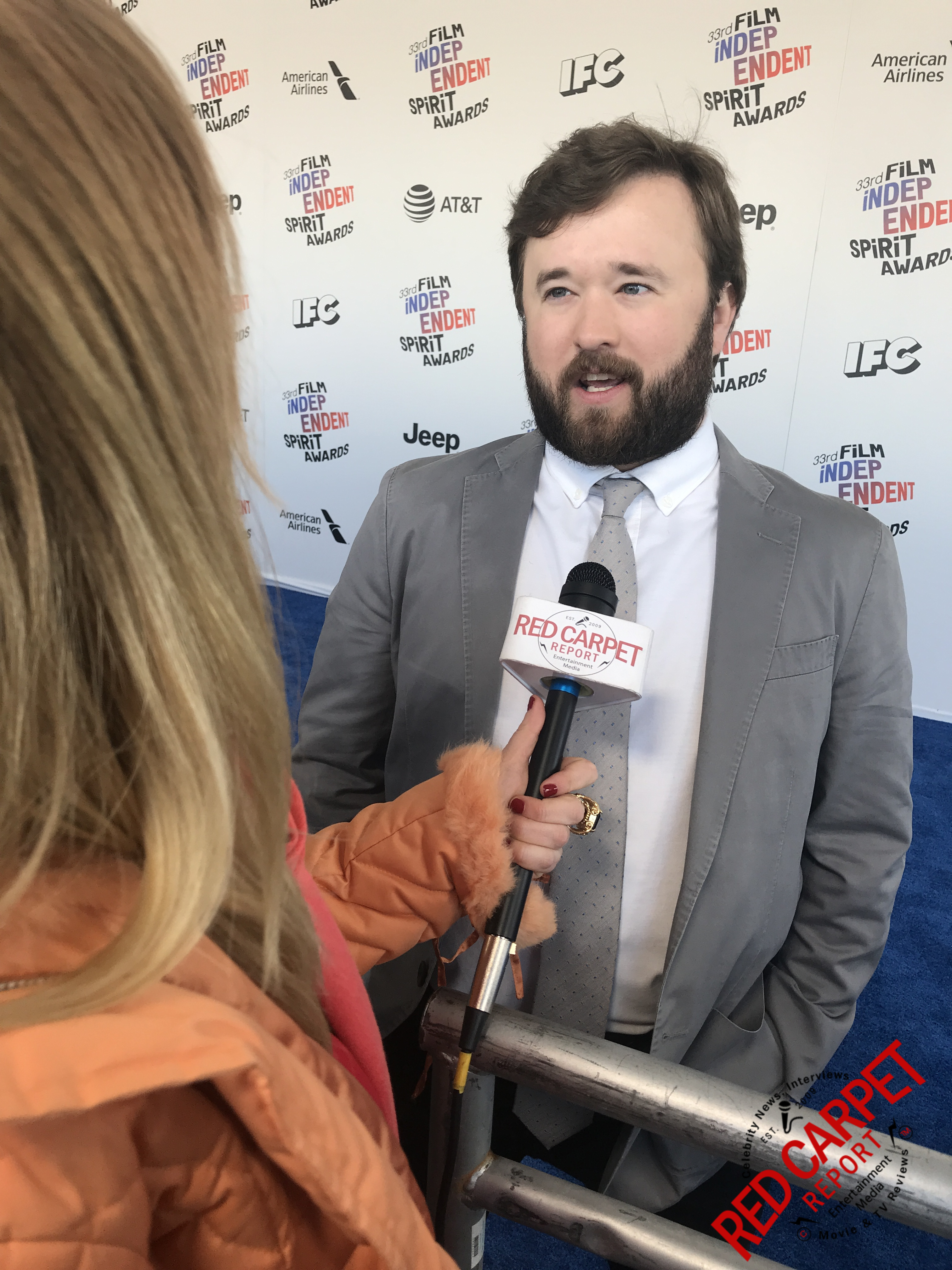The image captures a dynamic moment on the red carpet at an event, presumably the 33rd Film Independent Spirit Awards. The scene is viewed from a side profile, emphasizing the interaction between a female reporter and a middle-aged man being interviewed. The female reporter, identifiable by her blonde hair, holds a microphone in her left hand, extending it towards her interviewee. The microphone features a white inscription that reads, "Red Carpet Report." Her face is not fully visible in the shot due to the side angle. The man being interviewed is dressed in a sharp grey suit with a white shirt and a matching grey tie. He has brown hair and a well-groomed beard, exuding a poised and confident demeanor. The backdrop is filled with various logos and icons, prominently displaying "33rd Film Independent Spirit Awards," along with logos for AT&T and IFC. Additionally, there is a "Red Carpet Report" logo visible at the bottom right corner of the image, tying the scene together and emphasizing the event's media presence.